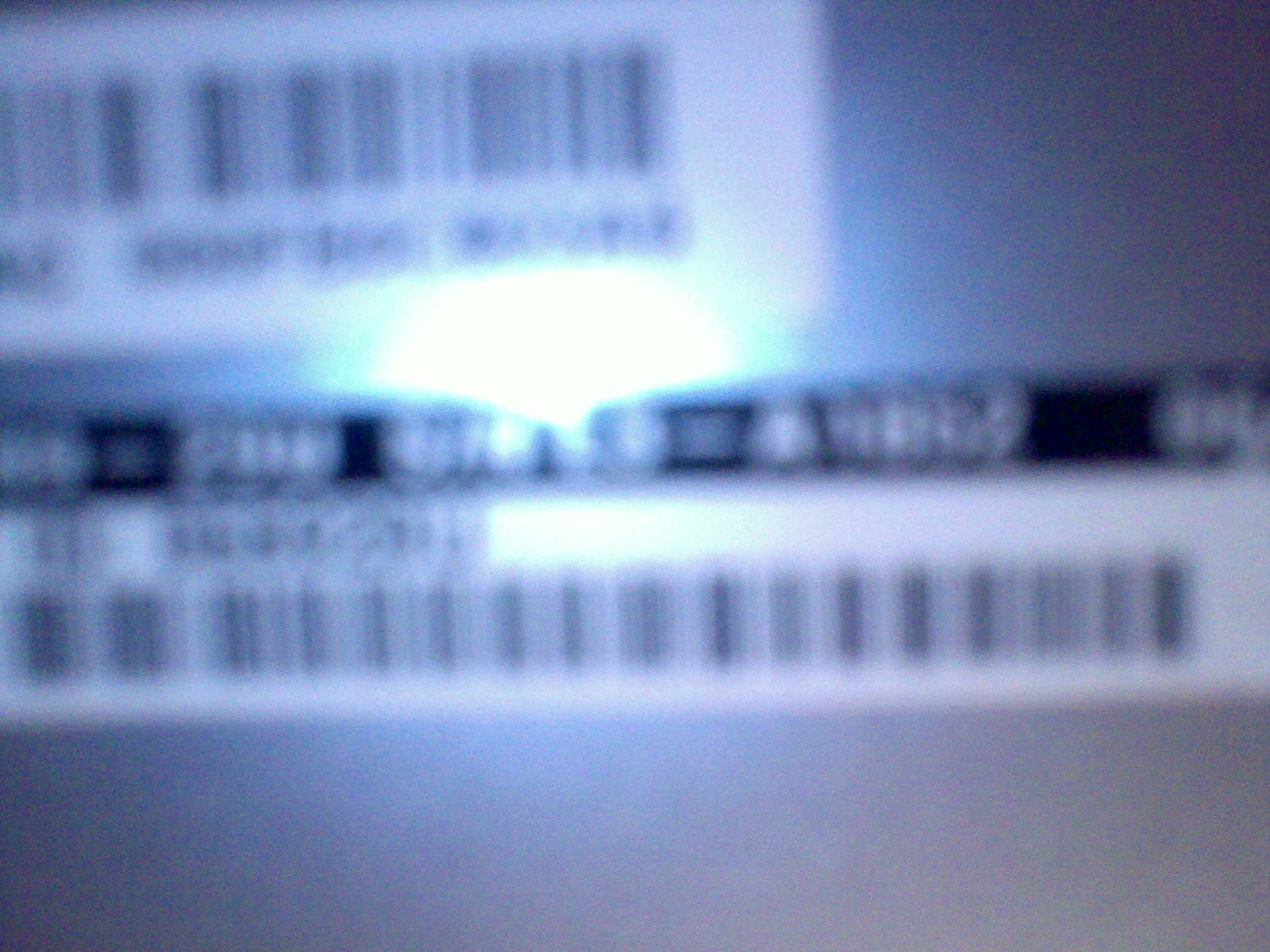An extremely out-of-focus photograph depicting a series of elongated barcodes set against various backgrounds. The bottom section of the image is dominated by a solid gray area, with a white stripe running horizontally near the top. This white strip features a nearly full-length barcode. A blue light subtly illuminates the center. Above the white barcode section, a black stripe with blurry, unintelligible numbers extends across. Roughly two-thirds from the left, another white bar, also adorned with a lengthy barcode, stretches most of the way across, accompanied by barely discernible text positioned just underneath it.